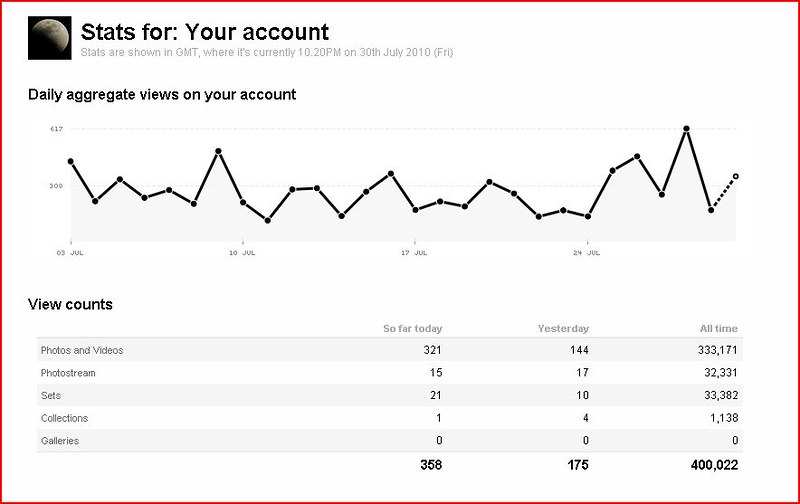The image depicts a screenshot taken from a webpage summarizing account statistics. At the top left corner, there's a small icon of a moon, next to text that reads "Stats for your account." Below it, in gray text, it states, "Stats are shown in GMT, where it's currently 10:20 PM on 30th July 2010, (Fri)." Following this, in bold black text, it says "Daily aggregate views on your account." Underneath, there is a line graph spanning from July 3rd to July 24th, illustrating daily views which peaked at 417 and a starting view count at 300. 

Below the graph, there's an informational table labeled "View Counts" which categorizes the data into "Photos and Videos," "Photo Stream," "Sets," "Collections," and "Galleries." The table shows views counted for today, yesterday, and all time totals. The details include the following counts:

- **Photos and Videos:** Today - 321, Yesterday - 144, All Time - 333,171.
- **Photo Stream:** Today - 15, Yesterday - 17, All Time - 32,331.
- **Sets:** Today - 21, Yesterday - 10, All Time - 33,382.
- **Collections:** Today - 1, Yesterday - 4, All Time - 1,138.
- **Galleries:** Today - 0, Yesterday - 0, All Time - 0.